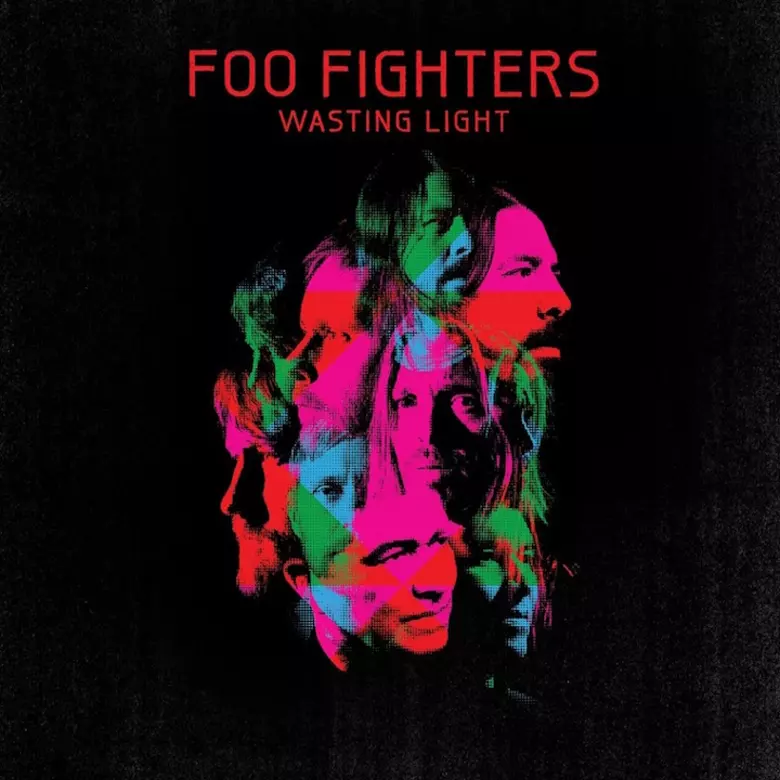This square image is likely the album cover for Foo Fighters' "Wasting Light." The cover features a pitch-black background that brings attention to the intricate details of the band members' faces, which are artistically stacked in a vertical column. The faces vary in size and orientation, with some looking left, others right, and some facing forward. The unique arrangement creates a dynamic visual effect. The title "Foo Fighters' Wasting Light" is prominently displayed in a vibrant pinkish-red font, adding a striking contrast to the somber background. The faces and heads are depicted in a mix of bluish-green, red, and pink tones, with hair rendered in lighter black and gray hues to distinguish it from the dark background. This contrasting use of color and positioning adds depth and visual interest to the album cover.